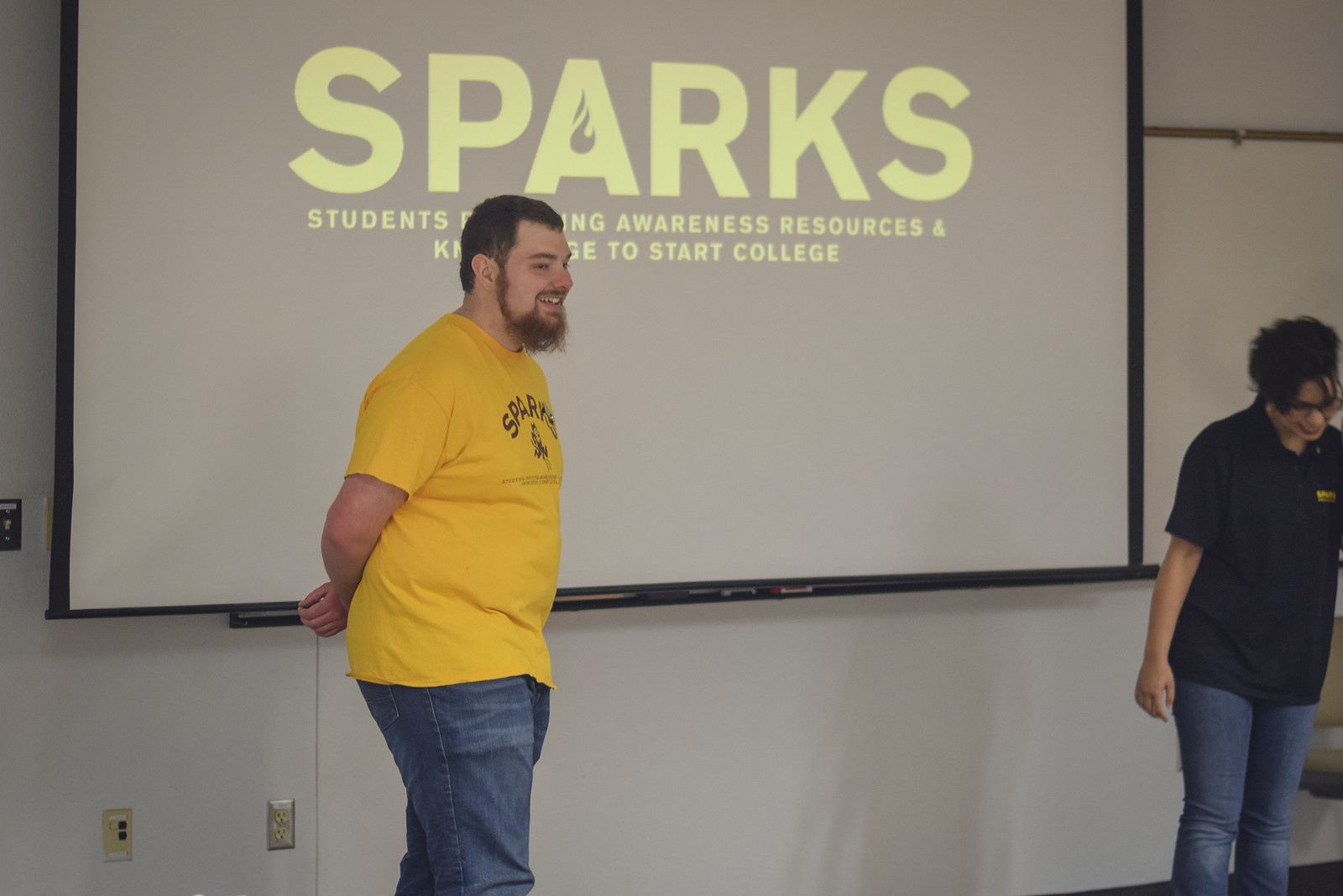In this indoor photo, two people are standing on a stage in front of a large whiteboard with a projection. The man on the left side has a short brown beard and hair, and he's wearing a yellow shirt with the word "SPARKS" emblazoned on it in capital letters, along with blue jeans. He has his hands behind his back and is standing confidently in front of the whiteboard, which displays the SPARKS logo and partially visible text: "Students," "Awareness," "Resources," and "To Start College." The woman's presence is noted on the right side of the whiteboard. She is wearing a dark blue shirt with a possibly small, yellow SPARKS logo and blue jeans, and she has glasses. She is looking down, and both individuals appear to be sharing a moment of laughter. The setting suggests they are giving a presentation about the SPARKS organization, likely at a community college, although the room itself is quite bare and unadorned.